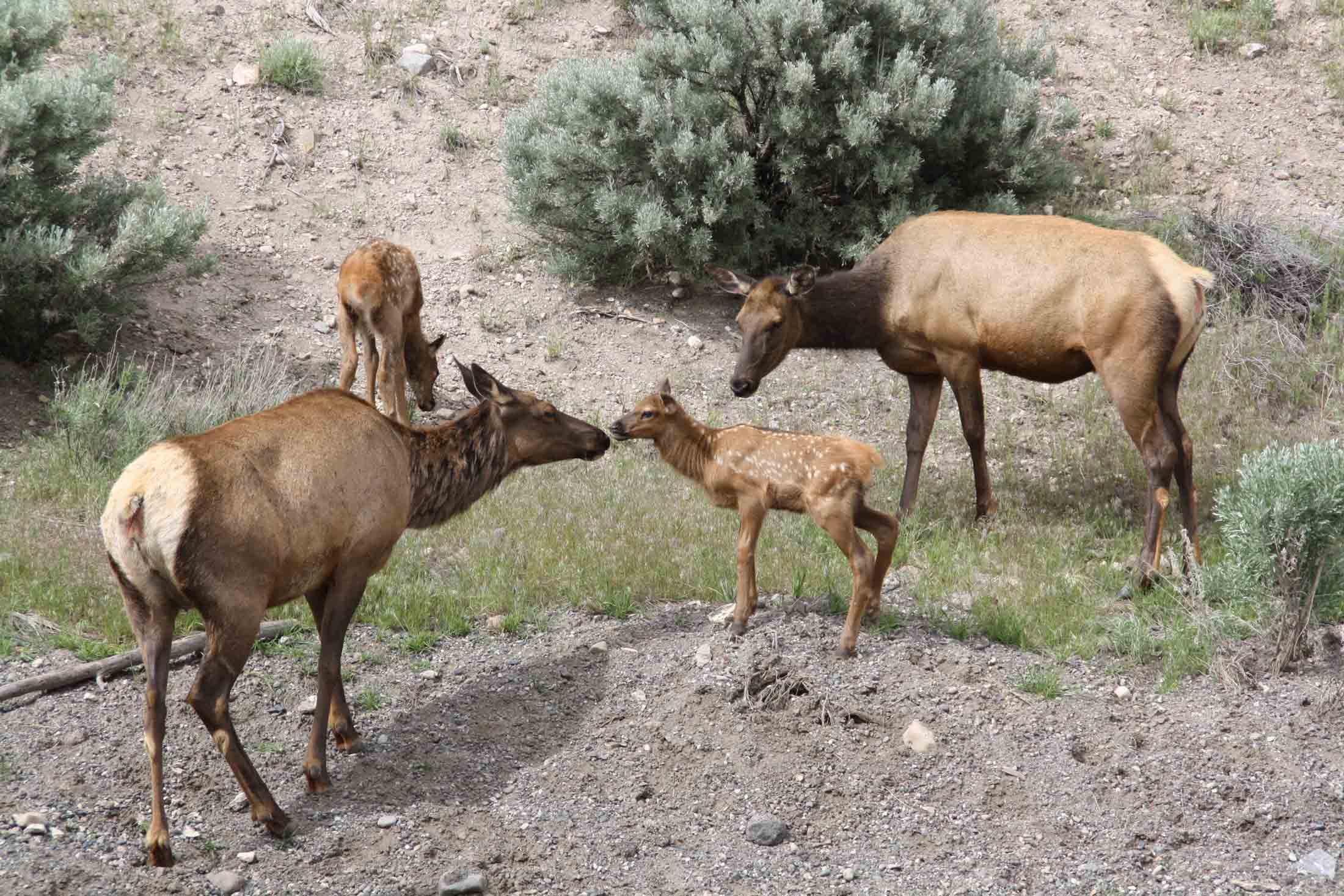In this landscape image, we see a serene scene featuring a family of four deer, likely consisting of two adults and two fawns, amidst a dusty and sparse mountain setting. The light brown and dark brown deer stand on a predominantly sandy and dirt-covered ground. The adults appear to be closely interacting with one of the fawns, while the other fawn stands slightly apart, seemingly engrossed in nibbling at some grass. The area is speckled with patches of sparse, green grass, some bushes, shrubs, and a few light green pine trees with hints of white, adding a delicate touch of color to the otherwise muted background. In the bottom right corner, a faint outline resembling a house logo can be observed, subtly blending into the sandy surroundings. The bottom left corner features darker dusty sand mixed with white pebbles, leading to the delicate legs and hooves of the nearest deer. The entire scene exudes a peaceful, family-oriented atmosphere, with each deer gracefully posed as they navigate their natural habitat.